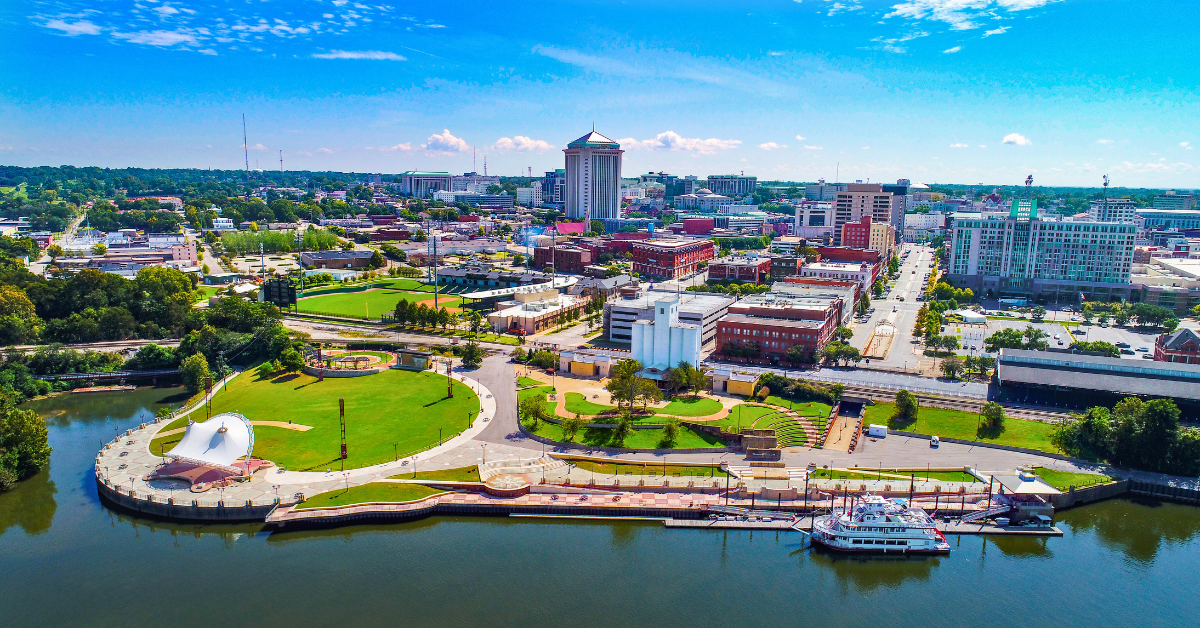This is a detailed aerial photograph, likely captured by a drone, showing a vibrant city by a large body of water on a bright sunny day. The expansive water space at the bottom of the image features a large ferry, or possible cruise boat, with numerous windows along its sides, and a paddleboat nearby. Adjacent to the water, there is a notable oval-shaped grassy area, surrounded by several content areas including shaded benches and what appear to be public restrooms. This leads to a prominent white building characterized by its three rectangular sections, the central one being the largest.

The city landscape behind this waterfront includes a mix of tall skyscrapers and smaller buildings, suggesting a blend of office spaces and apartments. The most striking building near the right-center of the image is a towering square structure capped with a triangular roof that features ornate red details, green accents, and a spire on top. The cityscape is dotted with lush green areas, including patches of grass, trees, and even a baseball field. The roads are bustling with cars, contributing to the lively urban atmosphere. The background is framed by a beautiful bright sky interspersed with white clouds, indicating it is the middle of a clear day.